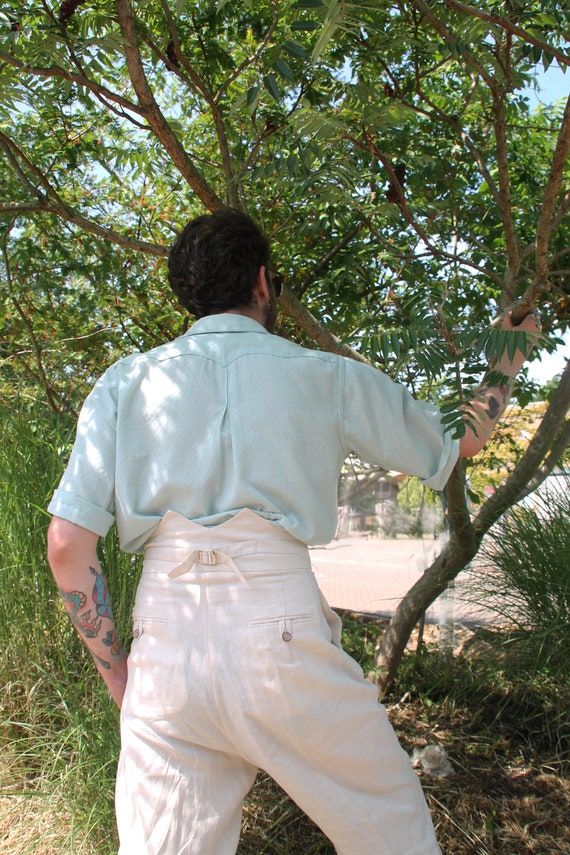In this photograph, a man is seen from the back, standing on the grass and holding onto a leafy green tree limb with his right hand. The man, sporting short black hair, sunglasses, and a beard, wears a light bluish-green shirt with rolled-up sleeves tucked into peculiar high-waisted white pants that tie in the back and have multiple cinch straps resembling those found on a backpack. His left arm is adorned with colorful tattoos, including a prominent octopus and another intricate design featuring red and turquoise shades. The scene around him is verdant, with lush green grass and an expanse of foliage. Across a red brick road behind him, there's a stone building with a tan roof, hinting at a street or possibly a lake area visible through the trees, all under a vibrant blue sky.